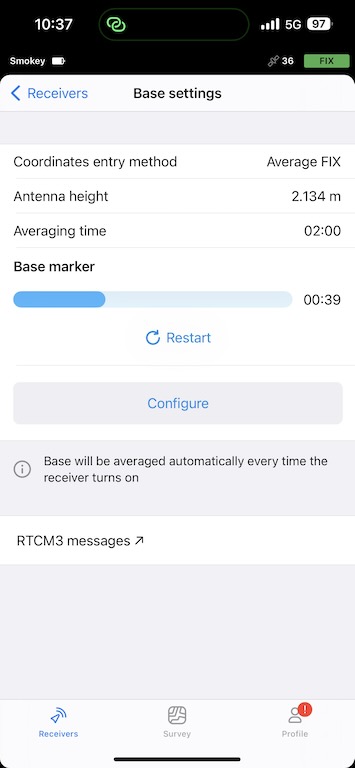The image depicts a screenshot from a mobile device interface. At the top, there is a black bar with white text details. The time displayed is 10:37. On the right side of this bar, there are icons showing a strong Wi-Fi signal, a "5G" network indicator, and the battery life at 97%.

Below the black bar, there is a search bar featuring an icon of two interconnected green links. Adjacent to this, the word "Smoky" is displayed along with a battery icon indicating a 36% battery level. Further to the right of this section, there is a green button labeled "Fix."

Beneath these elements, a pop-up window provides detailed information. The headings in this pop-up include "Receivers" and "Base Settings." Under "Base Settings," it specifies information such as:

- Coordinate Entry Method: Average Fix
- Antenna Height: 2.134 meters
- Averaging Time: 2 hours
- Base Marker: 39 seconds or 39 minutes

Additionally, there is a blue "Restart" button, and below it, a gray button with blue text that says "Configure." Towards the bottom of the pop-up, there is a note stating, "Base will be averaged automatically every time the receiver turns on."